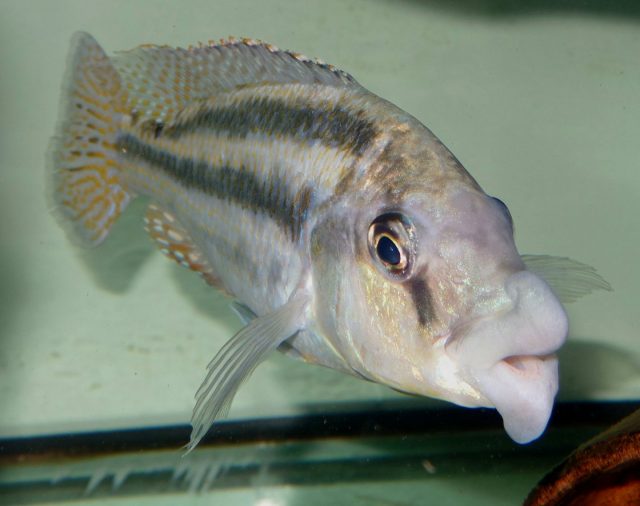This photograph captures a striking close-up of a medium-sized, golden-silver fish glistening as it swims in an aquarium. The fish, predominantly white with patches of brown and gold, exudes a shimmering effect under the light. It features large, distinct black eyes and big, white lips, which are open. The fish's body showcases two prominent black stripes running down its back, while its underbelly has subtle brown hues adorned with white specks. Its tail fin is short, exhibiting yellowish-gold stripes along with hints of black. Additionally, the fish has equally detailed dorsal and ventral fins that mirror the tail's color scheme. The photograph appears to have been taken within an aquarium, suggested by a possible glass background and the white backdrop likely being the aquarium wall, highlighting the fish as the focal point of the image.